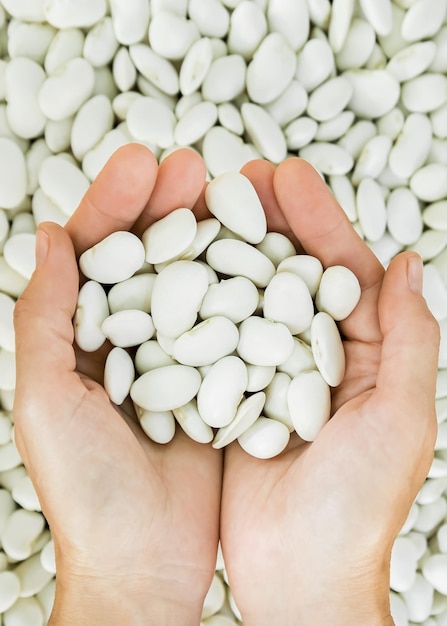A pair of Caucasian hands, cupped together, holds an abundant pile of light green lima beans, which nearly fill the hands halfway. The hands are positioned towards the center of the image, framing the beans prominently. These kidney-shaped beans have an off-white, eggshell green hue and appear smooth and slightly flat. In the background, the entire frame is filled with stacks of the same lima beans, creating a seamless backdrop that emphasizes the abundance of the beans. The foreground and background beans blend together, making the image rich with the texture and color of these light green legumes.